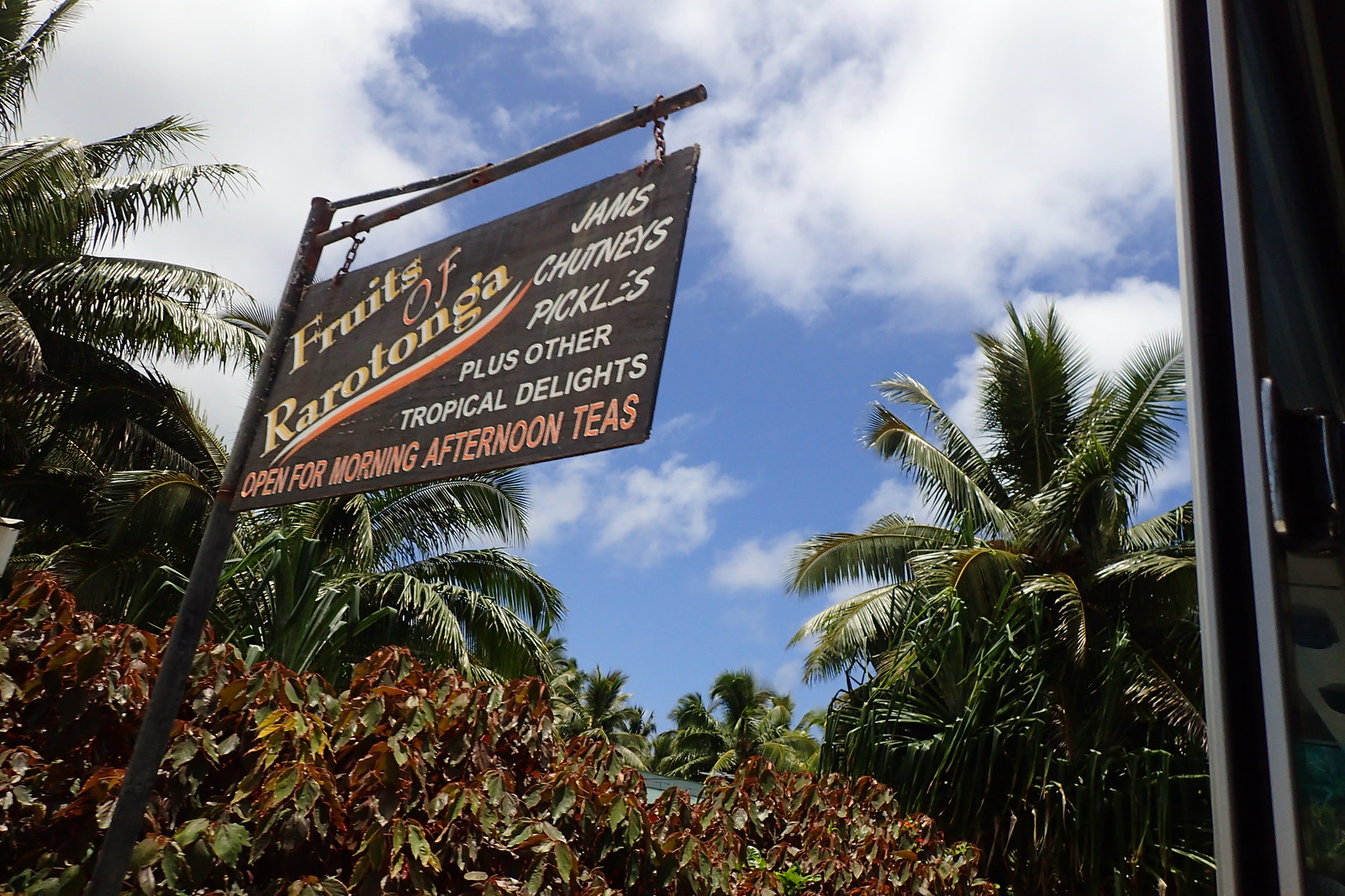The photograph captures an outdoor scene in a tropical area, dominated by a prominent rectangular sign that is viewed from below. The sign, affixed to a black pole and supported by a thinner black pole extending diagonally upwards, is positioned starting from the bottom left corner and extending towards the right side of the frame. Hanging by black chains, the sign has a black background and features the text: "Fruits of Rarotonga," in diagonal bold gold letters on the left side. The right side of the sign advertises in white, capital letters, "Jams, Chutneys, Pickles plus other tropical delights," and at the bottom, in orange capital letters, it reads, "Open for Morning Afternoon Teas." The background is filled with lush palm trees and a blue sky scattered with white clouds, enhancing the tropical ambiance. At the extreme right edge, there's a small visible section of what appears to be a sliding door, suggesting the location might be nearing a shop or café. The sign and its surroundings, including bushes at the bottom, suggest a vibrant setting possibly outside a local tea shop, set in the middle of the day with vivid tropical colors of blue, white, green, and various shades of brown and yellow.